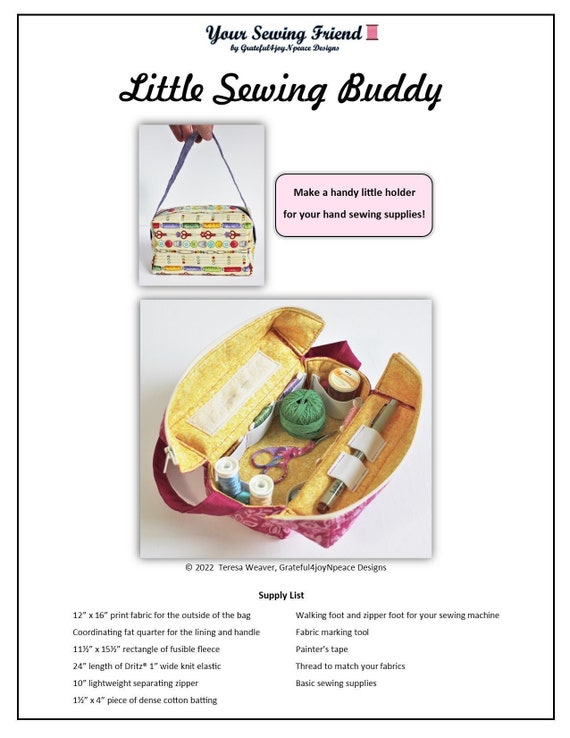The image is an advertisement for a product called "Little Sewing Buddy," by Grateful Enjoy Peace Designs. At the top of the ad, the bold text reads: "You're a Sewing Friend." Below it, in cursive, it says, "Little Sewing Buddy." The ad prominently features two photographs: one of the yellow, soft-sided sewing kit pouch with a handle, adorned with colorful designs of threads, scissors, and sewing tools. The pink rectangle text bar states, "Make a Handy Little Holder for Your Hand Sewing Supplies." The second photograph displays the Little Sewing Buddy opened up, revealing an organized interior with strapping to hold needles, marking pens, scissors, spools of thread, and various other sewing essentials. Additionally, there's a supply list at the bottom that details everything you'll need to create the Little Sewing Buddy, such as fabric, elastic, batting, a marking tool, painter's tape, matching thread, a zipper, and basic sewing supplies. The ad also includes a copyright note at the bottom: "Copyright 2022 Teresa Weaver."